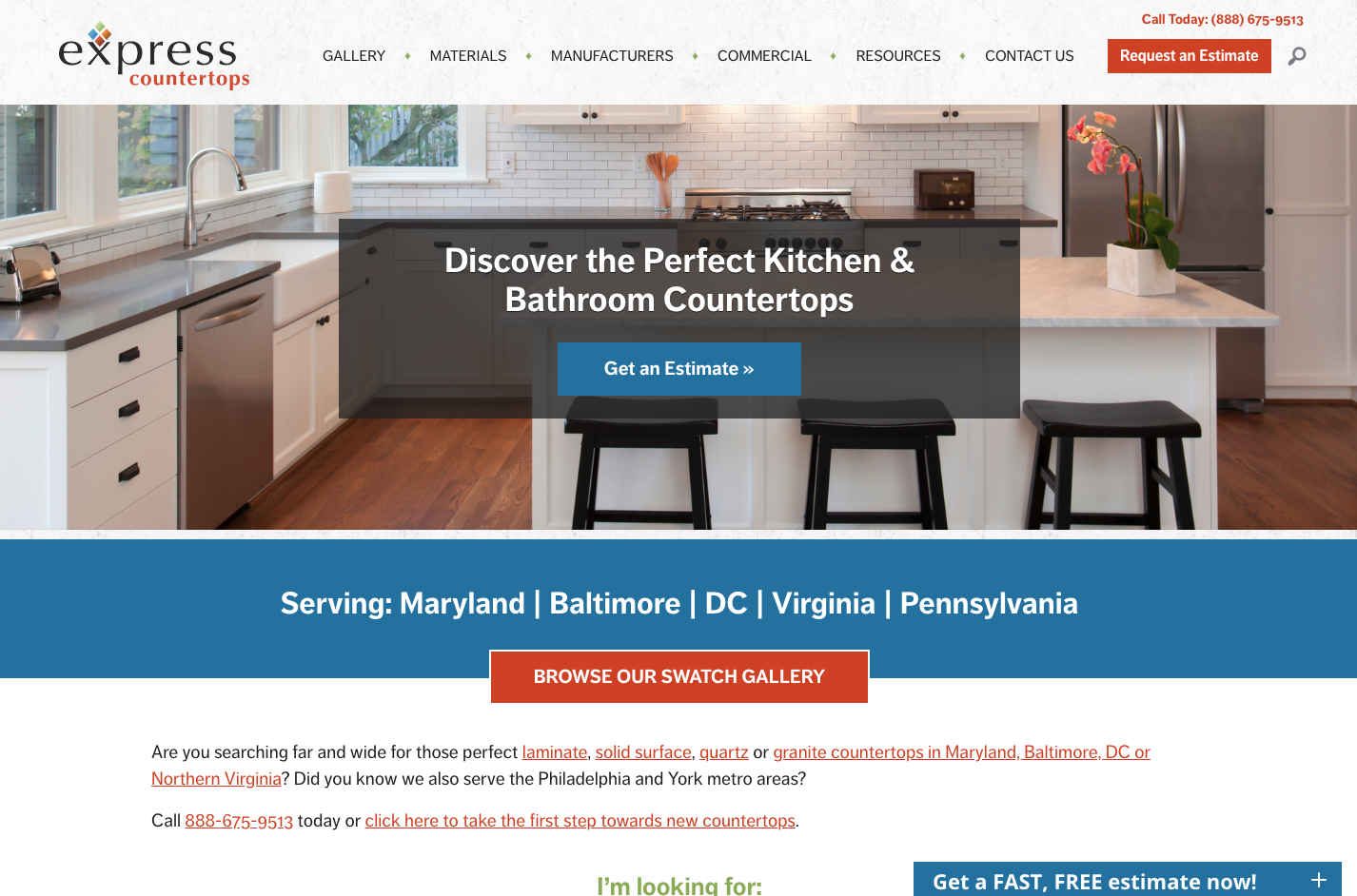"Discover the epitome of craftsmanship at Express Countertops, your go-to source for top-grade kitchen and bathroom countertops. The image showcases a pristine marble countertop with an integrated sink, perfectly complemented by a stunning tiled backsplash and sleek white cabinets. A trio of elegant seats provides a cozy dining space, while a state-of-the-art refrigerator ensures your culinary needs are met. The wooden flooring adds warmth, tying the elements together seamlessly. In addition, a large glass window frames a picturesque view of trees, bringing nature into your kitchen. The gallery features a diverse array of materials from premier manufacturers, offering comprehensive resources for your commercial needs. Dial 888-675-9513 to request an estimate or explore our collection of solid surfaces, laminates, and quartz options. Serving Maryland, Baltimore, D.C., Virginia, Pennsylvania, and beyond, we are committed to finding the perfect countertops for your space. Start your journey today and bring unmatched elegance to your home."